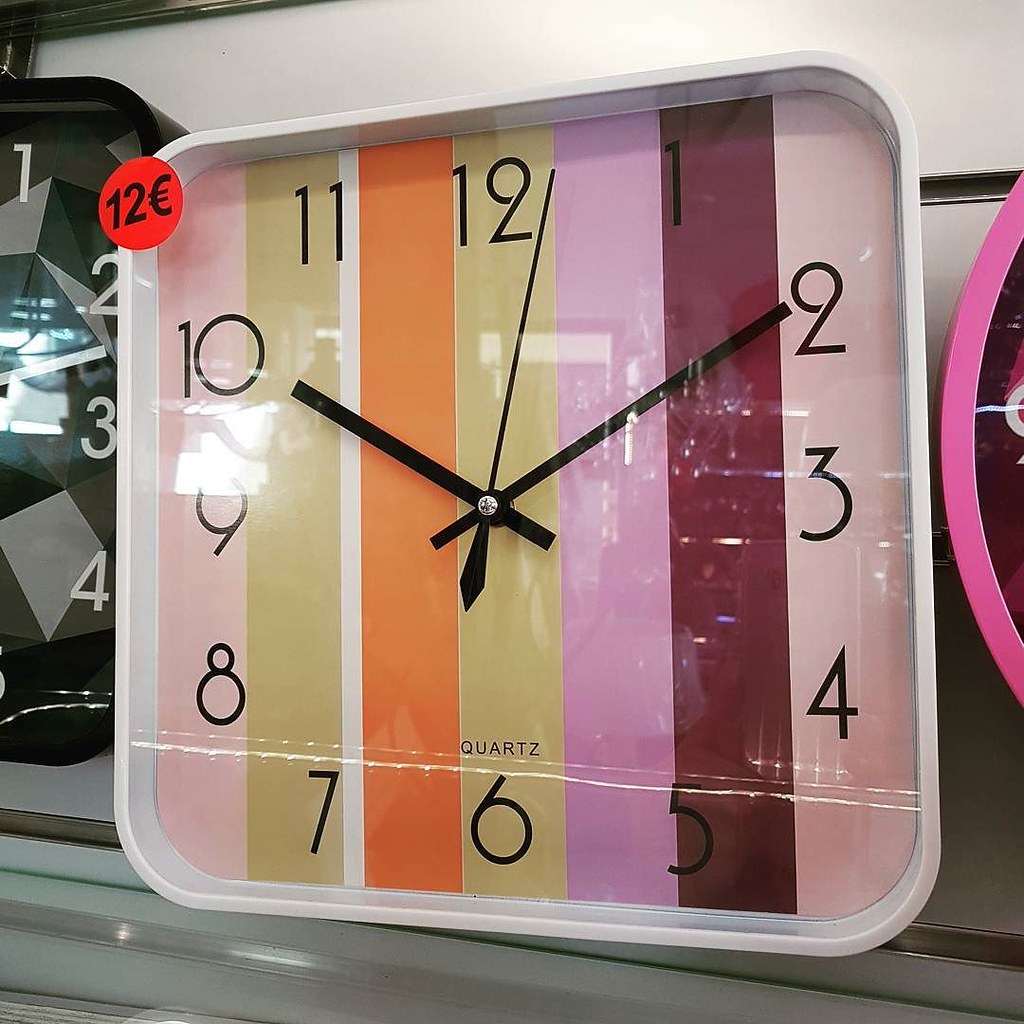In a retail store, a square clock takes center stage on a glass shelf with silver trim, set against a white wall accentuated by dark brown trim. The clock's outer frame is white, while the inner portion features vibrant stripes in colors such as pink, mustard, orange, green, lavender, maroon, and light pink. The clock hands point to 10:10, and "quartz" is inscribed on the face, which also includes all 12 numerals. Flanking this colorful timepiece, a black and white clock sits to the left, with the edge of a pink clock visible to the right, completing the eye-catching display.